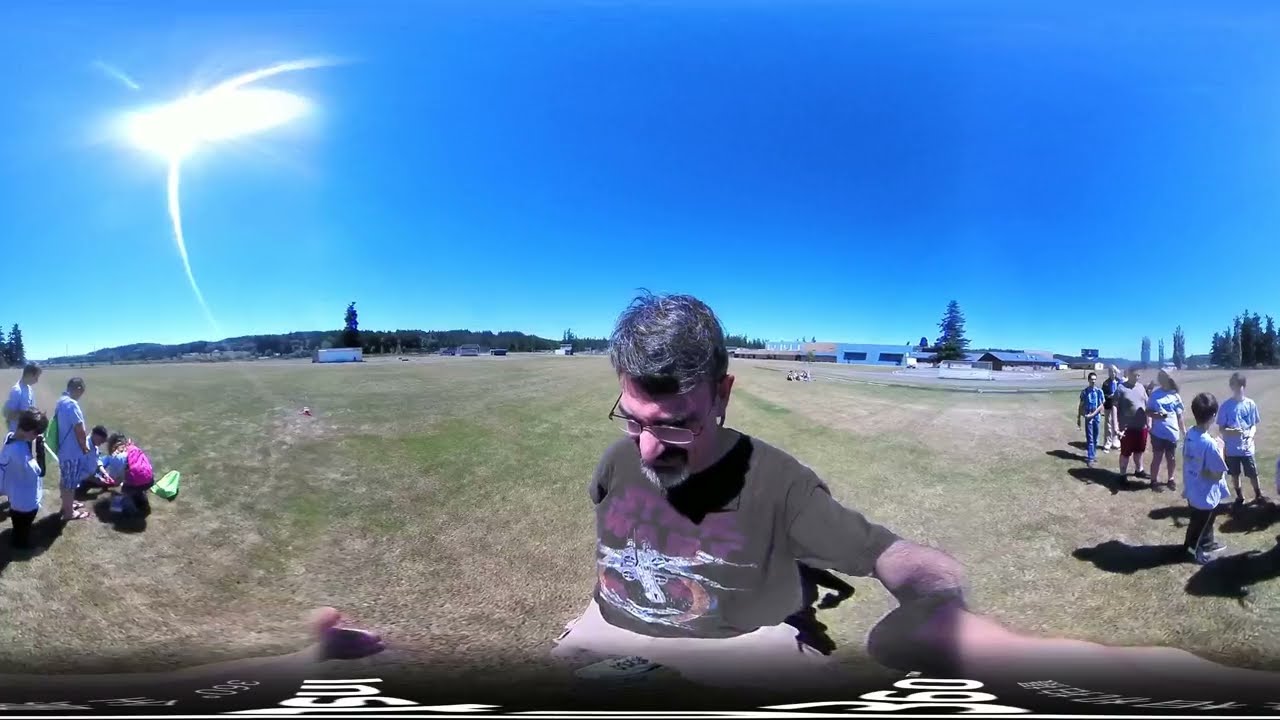In this clear, sunny outdoor panoramic image, numerous people are gathered on a large, flat grassy field flanked by clusters of trees on the horizon. To the right, a group of individuals stands, and to the left, another group, comprising both adults and children, is positioned with some standing and others kneeling. A central figure in the foreground—a bearded man wearing eyeglasses and a brown t-shirt with a design—is captured in a close-up, looking down, possibly holding the camera responsible for the image. Distantly, a taller church-like building and several lower structures are visible. The scene is bathed in daylight beneath a cloudless, intensely blue sky with a slight haze around the sun, creating distinct light streaks in the upper left corner. The setting suggests they're in a park, though this remains ambiguous, and the purpose of the gathering is unclear. The colors in the image include various shades of blue, green, and additional hues like yellow, pink, purple, black, and gray, contributing to a vibrant landscape.